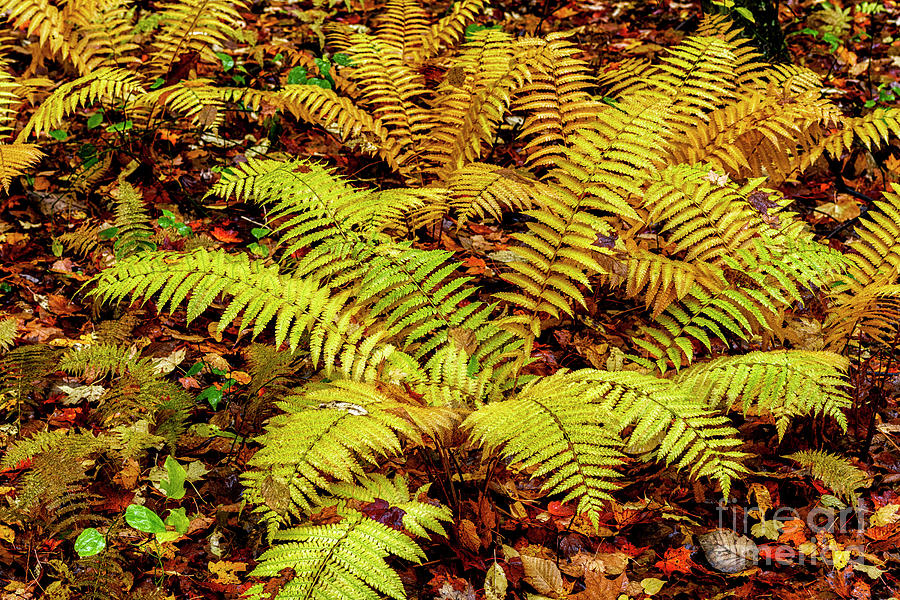This detailed, close-up nature photograph captures a scene dominated by light, intricate ferns growing low to the ground. The ferns, predominantly yellowish-green with hints of brown and light green, spread out their delicate, curving leaves from each stem. The main fern is centrally positioned, surrounded by smaller ones extending towards the left-hand corner, top, middle, and right edges of the image. The ground beneath and around these ferns is littered with fallen leaves in a variety of autumnal hues—brown, red, yellow, orange, and tan—indicating the fall season. The scene appears to be taken in wet conditions, possibly after rain or in the morning dew, lending a fresh, moist appearance to the foliage. In the bottom right corner, there's a watermark that partially reads "Fine Art," but the remaining text is unclear.